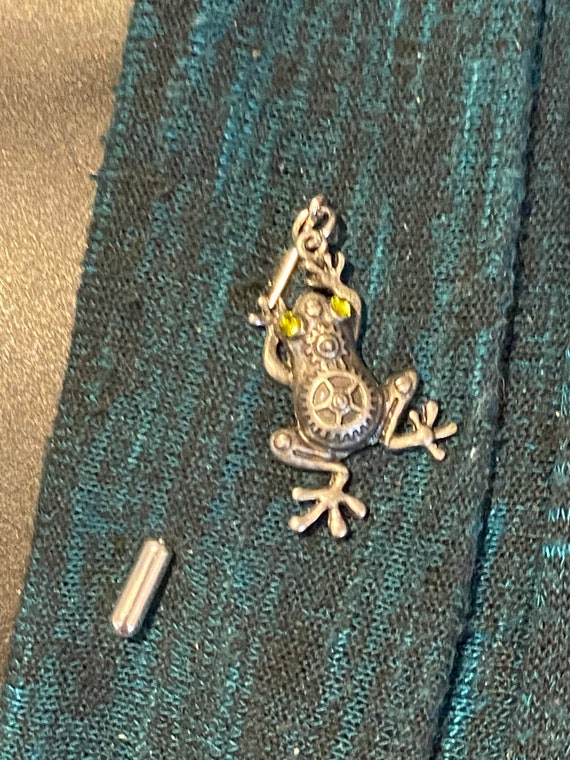This detailed close-up photograph captures a uniquely designed steampunk brooch, meticulously crafted in the shape of a frog. The brooch, positioned centrally in the image, is made of stainless steel, giving it a silvery appearance, with some descriptions hinting at hints of golden-bronze hues. The frog's design includes whimsical steampunk details, such as two gears on its back – a larger one on the bottom and a smaller one layered on top, evoking a clockwork aesthetic. The frog's legs are spread outwards, as if ready to pounce, and its striking eyes are adorned with yellow gemstones, contributing to its intriguing appearance. The brooch rests on a piece of fabric that features a mix of blue and black colors, although some interpretations suggest green and black or even blue and brown. Additionally, in the bottom left of the photograph, there is a small silver tube-like object, potentially part of the brooch or another element like a necklace, adding to the overall steampunk theme.